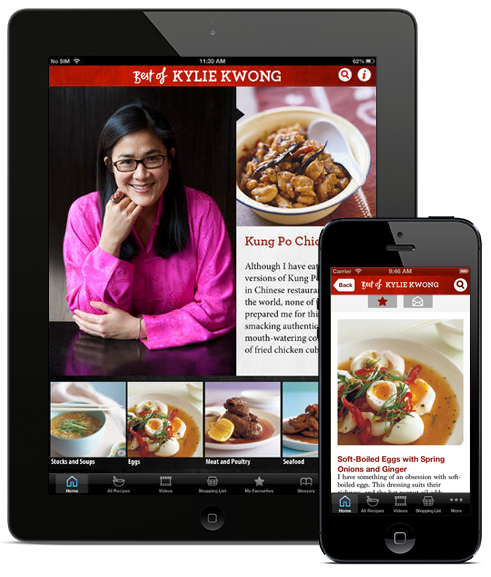The image showcases a webpage titled "Best of Kylie Kwong," prominently displayed in white letters on a red bar at the top of the page. The page is viewed on two devices: a tablet positioned centrally, and a smartphone to its lower right. Both devices are black, though the tablet appears to have a black or gray hue.

On the left side of the page background is black, transitioning to gray on the right. The main feature on the tablet's screen is a picture of Kylie Kwong, a woman with long, straight, shiny black hair and black glasses. She is dressed in a bright hot pink long-sleeve shirt. Her right hand is gently placed under her chin, while her left arm rests in front with her hand touching her right elbow. She is seated at a black table, capturing slight reflections of her pink clothing and hand.

To the right of Kylie Kwong's image, there is a vivid photograph of Kung Pao chicken served in a white bowl, set against a red and white tablecloth. Below this image, a red paragraph begins with the words "Kung Pao chick" before transitioning into a detailed text block describing the dish.

Beneath Kylie Kwong's portrait, the tablet displays four smaller images of different food items. The first image on the left shows a bowl of soup with white chopsticks laid across the top. It is labeled "Snacks and Soups" in white text. The adjacent image features a bowl of soup decorated with boiled eggs and red and green garnishes, accompanied by a label that reads "Eggs."

The same image of the boiled egg soup is also the principal display on the smartphone's screen. The text on the smartphone's screen describes it as "Soft boiled eggs with spring onions and ginger," written in red with subsequent descriptive black text below. The smartphone also features the red "Best of Kylie Kwong" banner at the top.

Returning to the tablet, to the right of the boiled egg soup photo, an image shows a brown dish with sauce and a slice of lemon, labeled "Meat and Poultry" in white on a black background. Finally, the rightmost image is a partially visible plate on a blue background labeled "Seafood."

This webpage offers a visually appealing and organized presentation of Kylie Kwong's culinary creations, accessible via both tablet and smartphone displays.